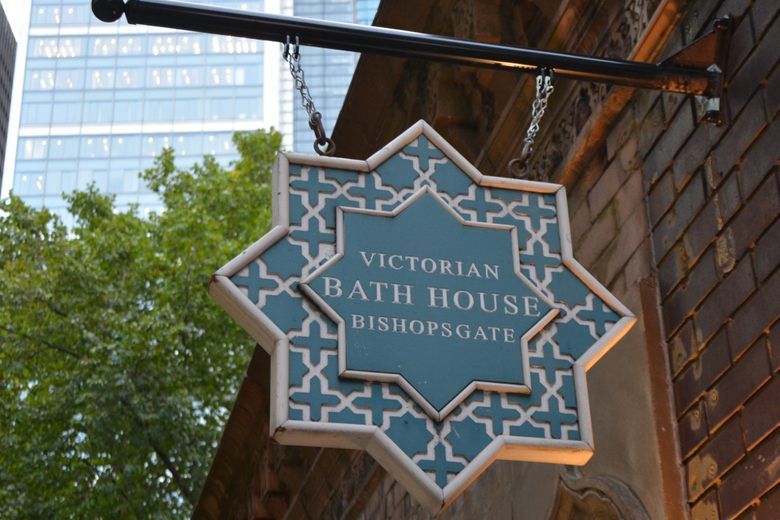The outdoor daytime photo captures an upward view of a sign extending from the side of a brown brick building. The skyward background showcases a tall skyscraper with numerous windows and a lush tree in full bloom with bright green leaves. On the right side, a black metal pipe protrudes horizontally from the building, suspending the sign with sturdy silver chains. The sign, designed as two interlocking squares forming an eight-pointed star, features a tan background with blue insets and borders decorated with blue crosses. Centrally, it prominently displays the text "Victorian Bath House, Bishopsgate" in tan. The harmonious contrast of the brown brick wall, the green tree, and the blue sky adds depth to the image.